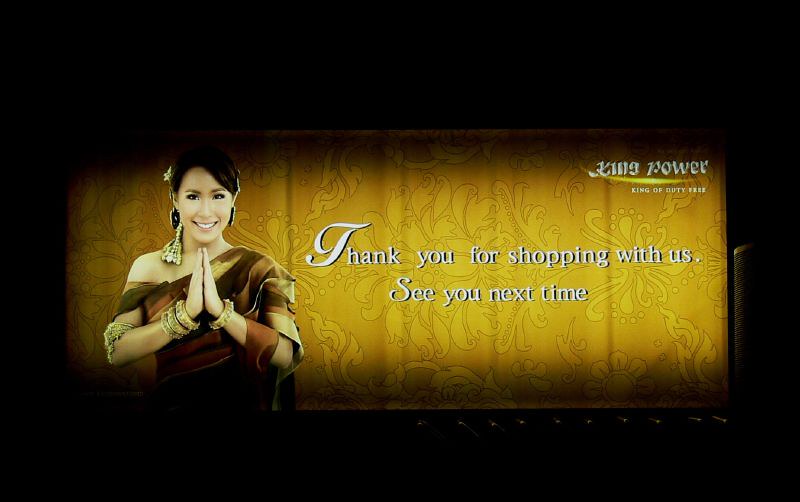The image features a dark black background with a rectangular golden-yellow central area that gradually fades darker towards the edges. Dominating the left side of this central area is a woman, possibly of Asian descent, adorned in a long, flowing dress that reveals one shoulder while draping over the other. She has dark brownish-black hair pulled into a bun and wears numerous gold bracelets on both wrists, along with long earrings and additional gold accessories on her arms. Her hands are positioned together under her chin in a gesture resembling a prayer or a thankful motion. Superimposed on the golden-yellow background are white letters that read, "Thank you for shopping with us. See you next time." Additionally, in the top right corner, the text "King Power" appears with a yellow slash beneath it, followed by the phrase "King of Duty," accompanied by some stylized characters. This combination of elements suggests the image is a promotional message from a store, expressing gratitude to customers.